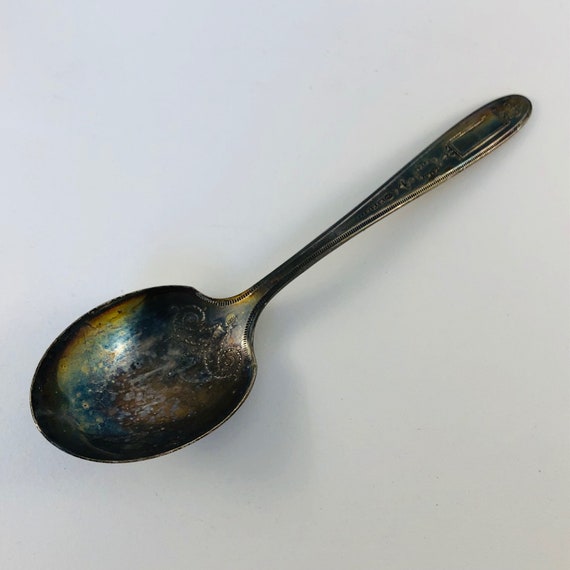This detailed color photograph captures a tarnished silver tablespoon placed indoors against a stark white surface, with the handle positioned in the upper right corner and the bowl angled toward the lower left. The back of the spoon features an intricate curlicue design that extends from the handle down to the bowl. The spoon’s surface shows signs of age and degradation, with discolorations ranging from black to blue, possibly due to heat exposure, reflecting the camera flash, and suggesting periods of neglect. Additional dark spots and blemishes further accentuate the spoon's weathered appearance. The spoon's tarnish and corrosion imply extensive wear, contributing to its antique look. The round handle tapers and then flares out as it meets the bowl. The spoon and its shadow dominate the centrally framed image.